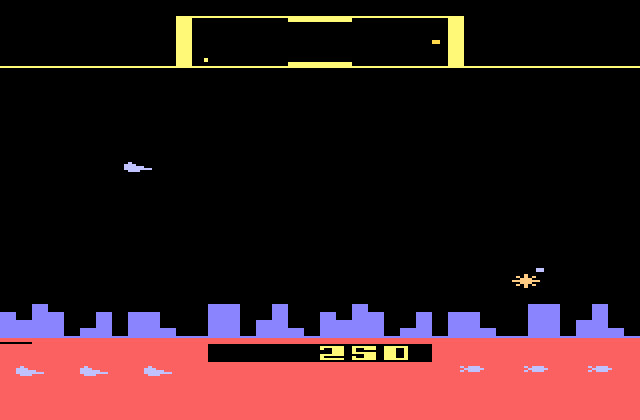This image is a screenshot of a vintage-style video game, reminiscent of those from the late 1970s to early 1980s. It features a blocky, retro airplane on the left side, flying towards the right against a black sky backdrop. Below, a city skyline is depicted with purple, two-dimensional rectangular buildings. Beneath the skyline, a red-hued landscape is populated with tank-like figures on the ground. A black bar runs across this red terrain, displaying yellow numbers that read "250," which appear to represent the player's score.